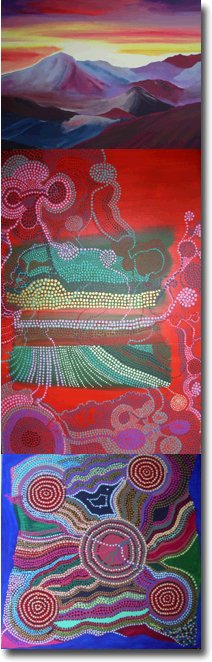The image is a vertically oriented, narrow composition consisting of three distinct pieces of mixed-media art arranged in a column. At the top is a meticulously detailed painting of a mountain range at sunset, featuring a vibrant sky that transitions through shades of yellow, orange, violet, purple, and red. Some mountains are majestically snow-capped, while others reveal rugged black rock. Below this, occupying the largest section, is an abstract artwork resembling an embroidered pillow. It has a striking red background with a central green area adorned with colorful beads in hues of yellow, green, darker green, and purple, arranged in dynamic swirls and patterns. The bottom section portrays another abstract piece, featuring a central circle flanked by four red and yellow bullseyes positioned at the corners. These elements are interconnected with wavy lines, creating a cohesive yet intricate design. A drop shadow effect unifies the trio, giving the impression of a singular, layered image.